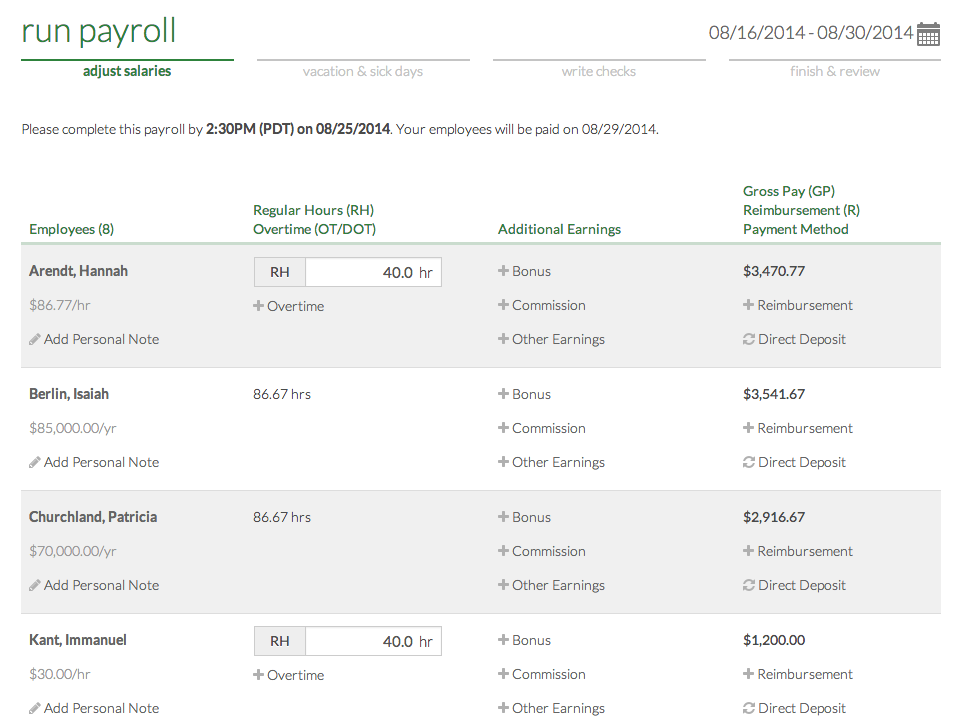This image showcases a payroll summary against a striking white background with two alternating rows of gray. The layout displays a gray row, followed by a white row, and repeats this pattern multiple times. At the top of the image, a clear, formal instruction reads: "Please complete this payroll by 2:30 p.m. PDT on 08-25-2014. Your employees will be paid on August 29, 2014."

Following this directive, there is a detailed list of employees, highlighting eight individuals. The table is divided into several columns: Regular Hours, Overtime Hours, Additional Earnings, Gross Pay, Reimbursement, and Payment Method. Here are some detailed entries:

1. **Hannah Airdent**:
   - **Hourly Rate**: $86.77
   - **Regular Hours**: 40
   - **Gross Pay**: $3,470.77

2. **Isaiah Berlin**:
   - **Annual Salary**: $85,000
   - **Hours Worked (This Pay Period)**: 86.67
   - **Gross Pay**: $3,541.67

3. **Patricia Churchland**:
   - **Annual Salary**: $70,000
   - **Hours Worked (This Pay Period)**: 86.67
   - **Gross Pay**: $2,916.67

Each row of the payroll summary is meticulously formatted to provide insightful details about employee earnings and related financial calculations for the particular pay period ending on August 25, 2014. This concise yet comprehensive payroll guide ensures clarity and accuracy in payroll processing and employee compensation.